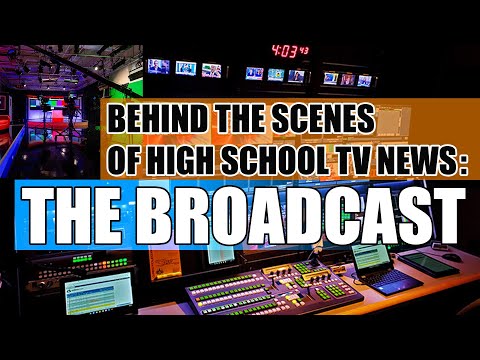The image is a detailed behind-the-scenes look at a high school TV news broadcast set. Dominated by a dark black background, the center features bold black text outlined in white on an orange backdrop reading, "Behind the scenes of high school TV news: The broadcast" in large white letters. Below this title, a mixing board, an open laptop, and several screens displaying live camera feeds are prominently placed, indicating their role in editing and adding sounds or videos. Above these elements, a row of monitors exhibits various scenes, possibly showing live or previously recorded footage. A digital timer at the top reads "403:48," and to the left, an equalizer is visible, with a bright, lit area likely representing the main set where the broadcasts are filmed. The detailed layout suggests a sophisticated setup, blending technology and media equipment essential for producing a high school news show.